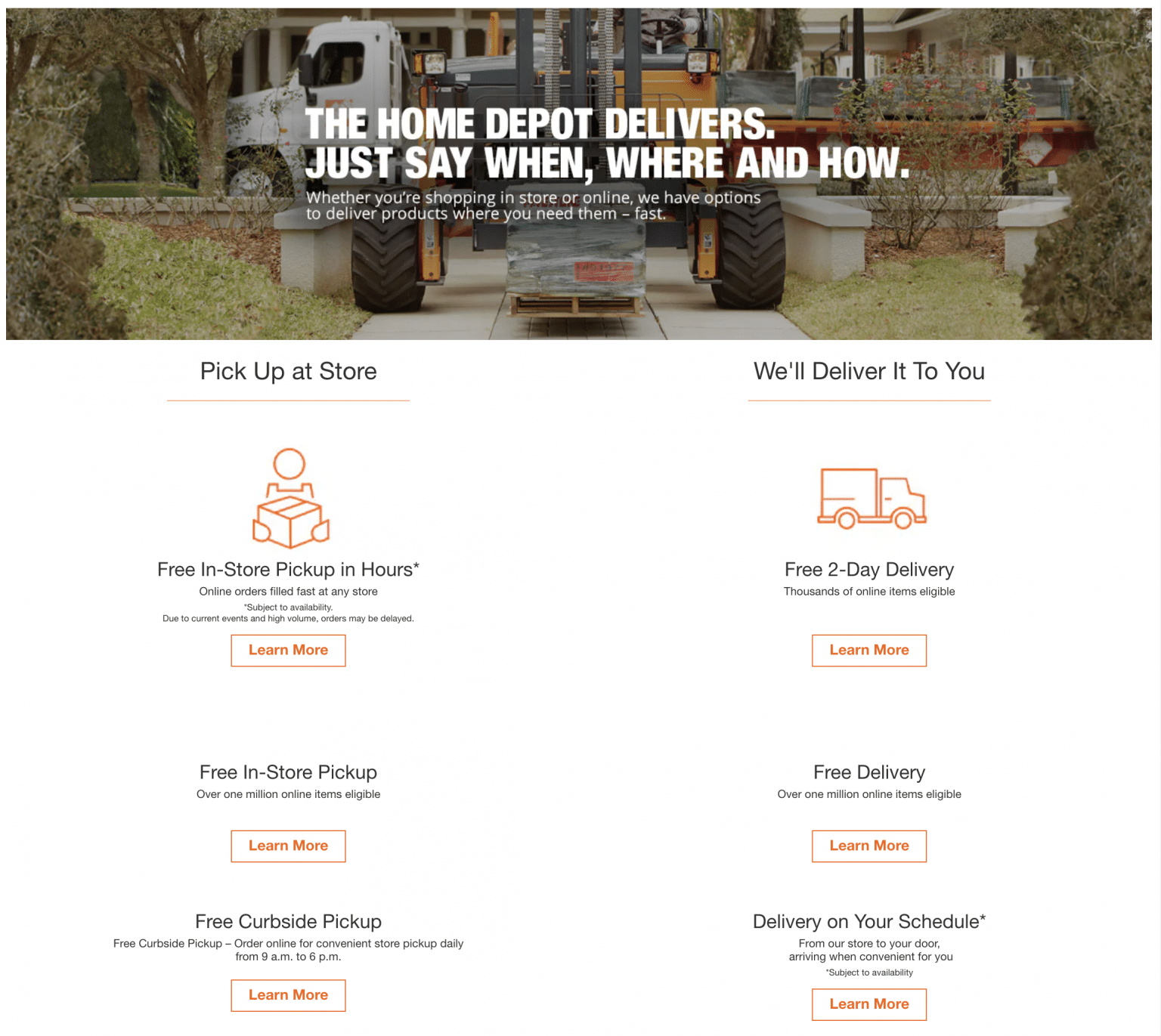**Detailed Caption:**

The image depicts a vibrant Home Depot advertisement focused on their delivery services. At the top, there is a picturesque outdoor landscaping scene featuring a white cab Home Depot delivery truck loaded with lumber. Adjacent to the truck, a tractor is actively unloading supplies from a pallet wrapped in plastic, set on a sidewalk flanked by lush lawns on both sides. A stone bench wraps gracefully around a tree or plant, adding a touch of natural beauty to the scene.

Prominently displayed in bold white block lettering, the ad reads: "The Home Depot delivers, just say when, where, and how." Beneath this, a smaller white font states, "Whether you're shopping in store or online, we have options to deliver products where you need them fast."

Below the image, the ad details various pickup and delivery options. On the left-hand side:
- **Pick Up at Store:** Accompanied by an orange line, this section features an orange stick figure holding a box with the text "Free in store, pick up in hours" in black. Further explanation in black says, "Online orders filled at any store, subject to availability. Due to current events and high volume, orders may be delayed." Below, an orange box invites viewers to "Learn more."
- Following this, another black text line mentions, "Free in store pick up, over 1 million online items eligible," with a subsequent orange box labeled "Learn more."

Continuing below:
- **Free Curbside Pickup:** It explains, "Order online for convenience, store pickup daily from 9am to 6pm" in black, followed by an orange box stating "Learn more."

On the right-hand side, under the image:
- An orange truck icon accompanies the phrase "We'll deliver it to you" with a corresponding orange line underneath.
- **Free Two-Day Delivery:** Described in black, "Thousands of online items available, eligible," followed by an orange box with "Learn more."
- Further in black text: "Free delivery, over 1 million online items eligible," with another "Learn more" in an orange box.
- Finally, "Delivery on your schedule from our store to your door, arriving when convenient for you, subject to availability" in black, capped off with an orange box stating "Learn more."

This comprehensive ad encapsulates Home Depot's commitment to providing flexible and efficient delivery and pickup options for their customers.